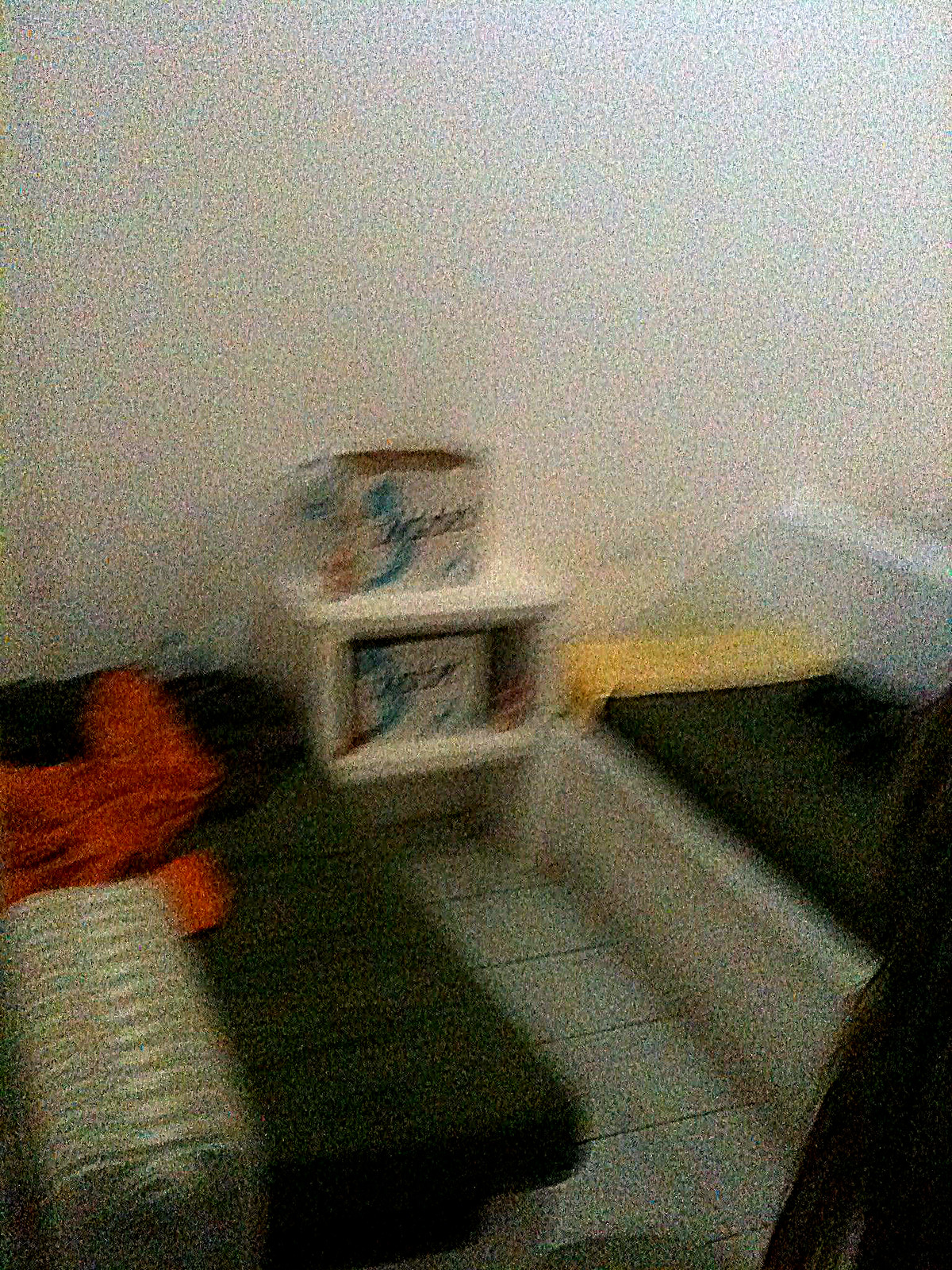The image shows a blurry and distorted photograph of an indoor room with white or off-white walls. In the center, against the wall, stands a white wooden end table or small shelf. On top of this table is a white box with teal lines or curves, and an identical box is placed on a shelf within the table. There may also be a water bottle on the table. To the left, there's what appears to be a futon or couch with a red piece of clothing draped over it. Directly opposite, on the right side of the image, is a white wooden seating area with a dark-colored cushion and a yellow item of clothing. The floor in the middle is tiled, and there seems to be a long, skinny mattress laid out on another ledge, likely another bench. In the bottom left corner is a radiator, while the bottom right corner is obscured by a black blob. The room appears to be quite standard but is challenging to discern due to the grainy quality of the photo.